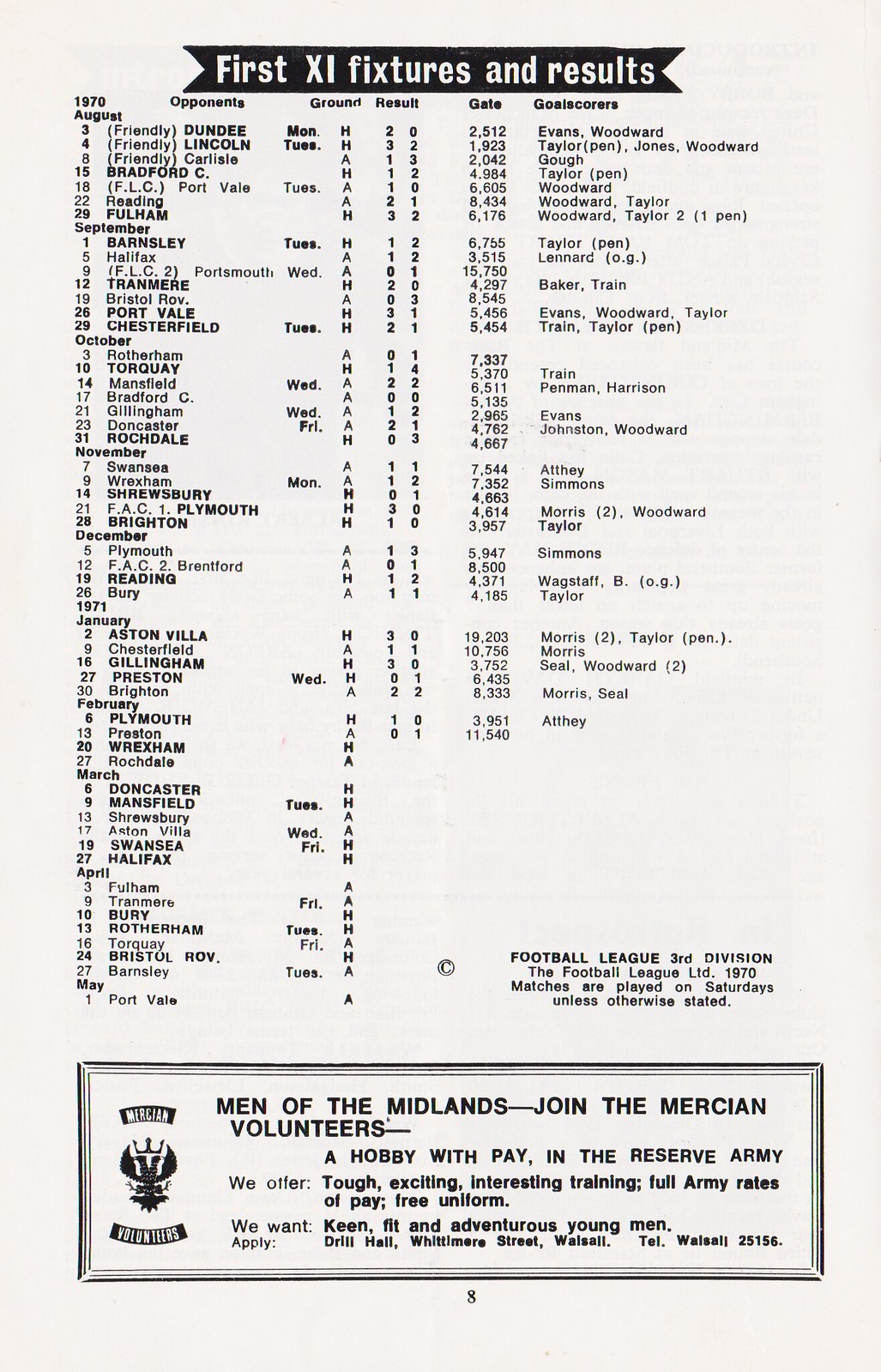The image is a page that appears to be from a football league brochure or magazine, dating back to 1970. At the top, a prominent black banner states "First XI Fixtures and Results." The page is organized into six columns labeled "1970 August," "Opponents,” "Ground,” "Result,” "Gate,” and "Goal Scores.” Specifically, the entry for August 7 lists a friendly match against Dundee, held on a Monday, with a resulting score of 2-0, attended by 2,512 spectators, and Evan Woodward among the goal scorers. Mid-page results continue consistently with a line of results approximately halfway down, stopping about three-quarters of the way through the column. Toward the bottom right, text notes "Football League, 3rd Division, The Football League Limited, 1970," and mentions that matches are played on Saturdays unless stated otherwise. In the lower section is an advertisement within a square, promoting the "Men of Midlands" for joining the Mercian Volunteers in the Reserve Army, offering tough, exciting training and full Army rates of pay, encouraging keen, fit, and adventurous young men to apply. The overall design is black text on a white background, with clean, vertical alignment of columns and a structured presentation typical of informative pamphlets or brochures related to football league data and army recruitment.